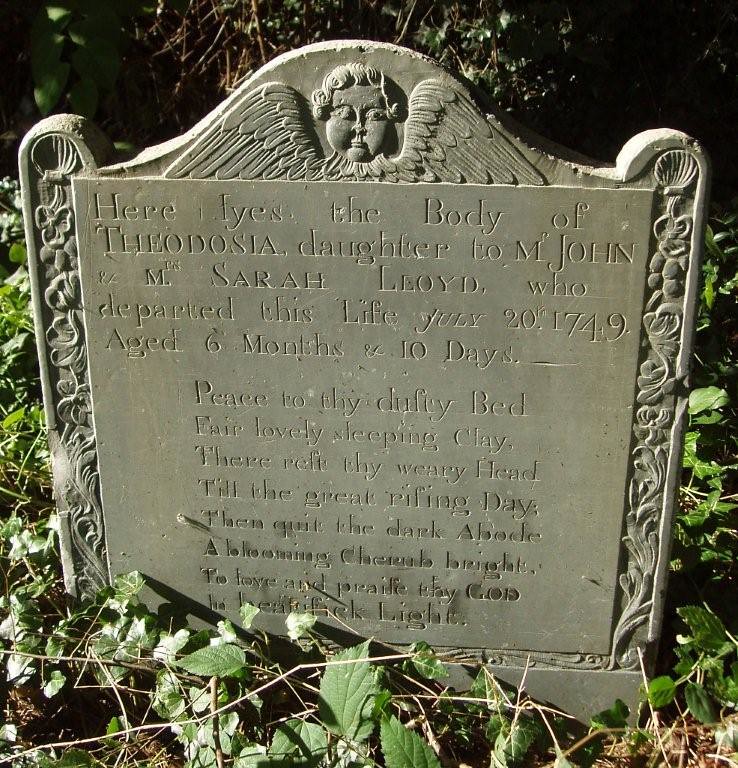This photograph captures an ornate stone tombstone partially obscured by leaves and small plants in the foreground and background. The tombstone features intricate designs along its sides, including motifs of shells and perhaps waves or flowers, culminating in a carved baby angel with wings and curly hair at the top. The epitaph reads, "Here lies the body of Theodosia, daughter of M. John and M. Sarah Lloyd, who departed this life July 20th, 1749, aged six months and ten days." Below this, an eight-line poem begins with "Peace to thy dutily bed, fair lovely sleeping clay, there rests thy weary head," though the lower portion of the text is difficult to decipher due to dirt and aging. The photograph looks down at the headstone, highlighting its aged beauty and the natural elements encroaching upon it.